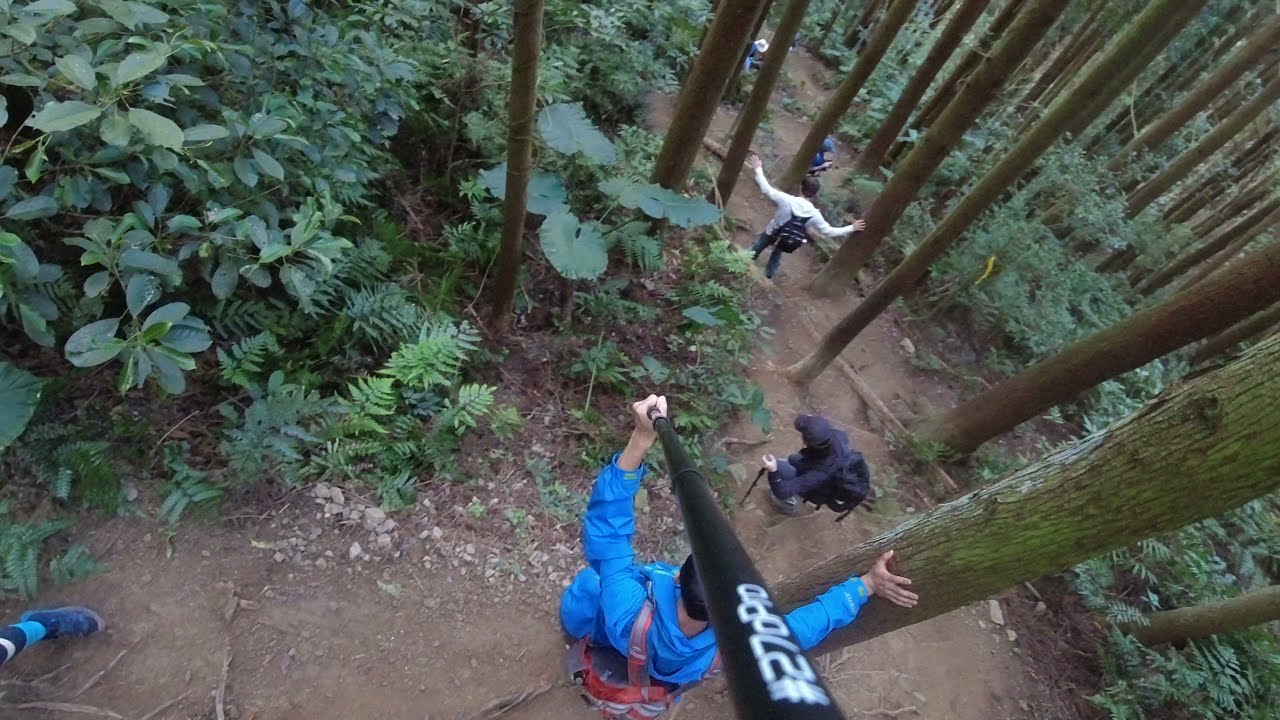In this aerial photograph taken in a wooded forest, the scene is densely populated with slender trees adorned with brownish-green moss. The image is rich with vibrant colors, including shades of green, blue, black, white, brown, and tan. The forest floor is dominated by a winding dirt path made of dark soil, meandering from the bottom left corner towards the center of the image, and further up to the top. 

Several people are captured along this trail. Closest to the center is an individual holding what appears to be a stick or a bat-like object. This person, clad in a blue hoodie and a backpack with red highlights, has their right hand resting on a tree beside them. To their right, a person dressed in black appears to be kneeling or squatting. 

Further up the trail stands another person in a white hoodie, balancing with outstretched hands. They are wearing a black backpack and seem to be navigating the uneven terrain. In the background, just to the left of center, another figure is partially hidden by a tree, seemingly absorbed by a phone. Beyond them, a faint outline of yet another person is visible, strolling along the path.

The lower left corner of the image reveals the blue shoe and sock of yet another individual, emphasizing the crowded and lively atmosphere of the forest trail. Surrounding the path and characters are various plants, including large-leaved bushes on the upper left and patches of suspected poison ivy and ferns scattered throughout.